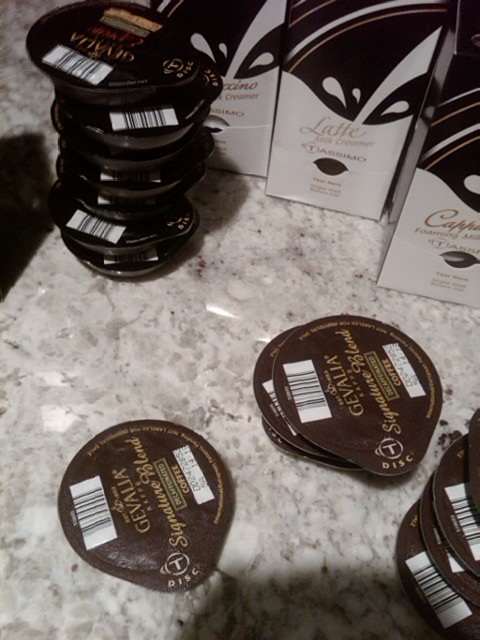The image showcases a kitchen countertop viewed from a sharp 45-degree downward angle. The countertop has a speckled design, predominantly light grey with specks of different shades of grey and black, giving it a marble-like appearance. Scattered across the countertop are coffee pods used for a coffee machine, each featuring a dark brown surface with goldish-yellow writing. Notable markings on the pods include a T inside a circle with the word "DISC" beneath it, along with visible barcodes. In the foreground, there is a single coffee pod on the left, a stack of three pods to the right, and another stack of four or more pods extending out of the frame at the bottom right. Behind these, more coffee pods and boxes are aligned, displaying the same T stripe logo found on the pods. The boxes are identified by different labels such as "cappuccino," "latte," and "creamer," suggesting a variety of coffee-related products. Additionally, the lighting casts a convex arc of shadow from the photographer into the foreground, adding to the depth of the scene.